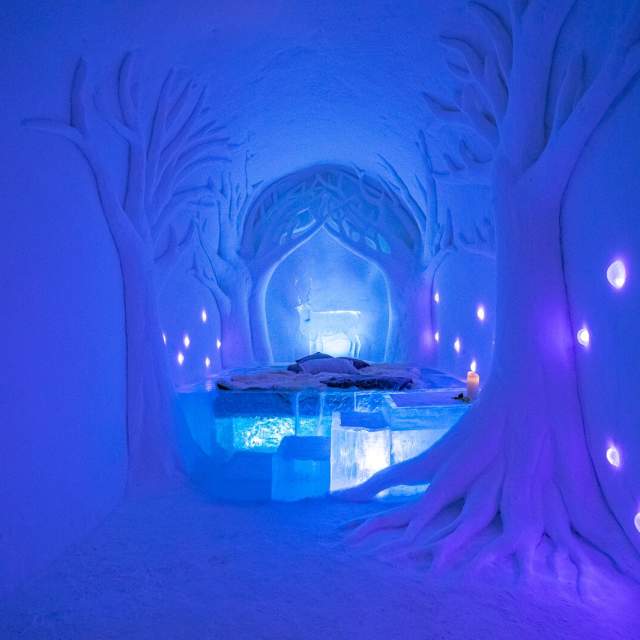This image depicts a mesmerizing ice-themed hotel room that resembles an intricately carved ice cave. The centerpiece of the room is a bed crafted from a solid block of ice, adorned with fluffy blue blankets and pillows. The base of the bed features subtle internal lighting, shining through the ice, creating a magical glow.

Flanking the bed, the walls and floor are bathed in a mix of deep blue and purple lights, enhancing the cave's ethereal ambiance. On either side of the cave room, exquisite carvings of trees without leaves stretch upward, their bare branches arching gracefully.

Situated against the back wall is an ice sculpture of a majestic stag with impressive antlers, backlit to create a soft, luminescent effect. The stag appears to be standing on a small ice ledge, and to its right, a candle lit in a warm red hue adds a touch of cozy warmth to the otherwise cool palette of the room.

Further enhancing the scene are small white dome lights embedded between the tree carvings along both sides of the room, contributing to the overall dreamlike atmosphere. This exquisite ice room, with its enchanting blue glow and exquisite details, offers a captivating blend of nature and fantasy.